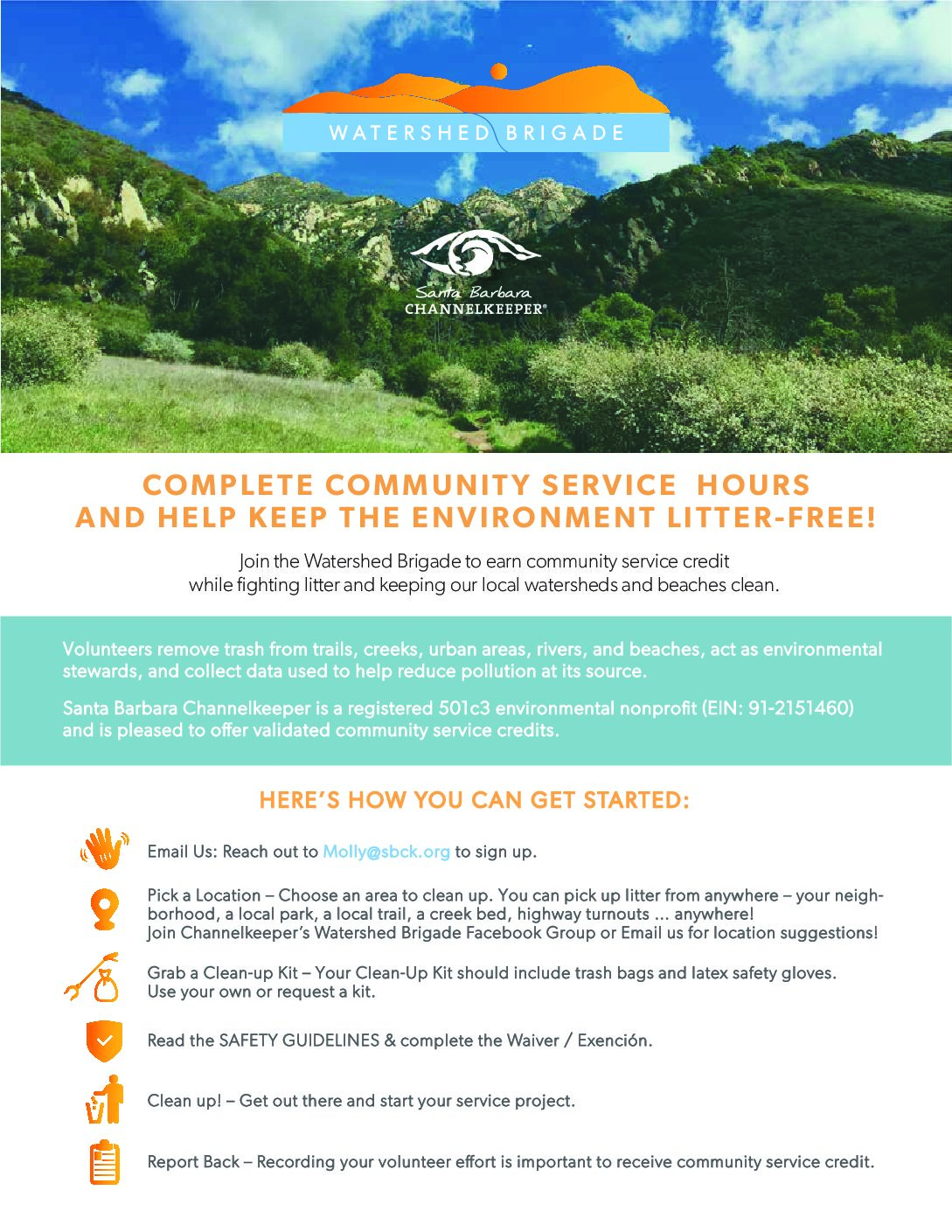The image features a detailed and vibrant poster promoting the Watershed Brigade initiative by the Santa Barbara Channel Keeper. At the top, set against a clear blue sky with floating clouds, a prominent orange-colored mountain logo catches the eye, followed by the bold title "Watershed Brigade" printed on a blue rectangle. Beneath this, the Santa Barbara Channel Keeper logo is displayed, characterized by a design resembling an eye. 

The scene depicted includes verdant rolling hills with bright green grass, portraying a lush, natural environment. The heading underneath reads "Complete Community Service Hours and Help Keep the Environment Litter Free," inviting volunteers to join the Watershed Brigade for community service credits while protecting local watersheds and bridges through litter removal.

Details are provided on how to get involved: 
1. **Email Us**: Reach out to molly@sbck.org to sign up.
2. **Pick a Location**: Options include neighborhoods, parks, trails, creek beds, and more, with support from the Brigade's Facebook group for suggestions.
3. **Grab a Cleanup Kit**: Assemble a kit with trash bags and safety gloves, either your own or requested.
4. **Read Safety Guidelines**: Complete the necessary waiver or exemption forms.
5. **Clean Up**: Initiate your service project.
6. **Report Back**: Recording your efforts is vital for obtaining community service credits.

The Santa Barbara Channel Keeper, a registered 501(c)(3) environmental non-profit (EIN: 91-2151-460), supports this initiative to empower environmental stewardship and combat pollution at its source.